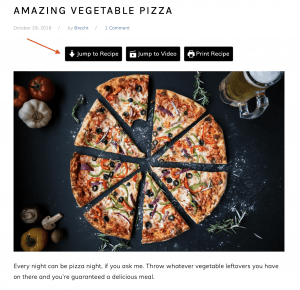A small image capture is promoting a delectable vegetable pizza. In the upper left corner, the text reads "Amazing Vegetable Pizza." The top of the image features three rectangular icons, each with red arrows pointing diagonally towards them. These icons are labeled "Jump to Recipe," "Jump to Video," and "Print Recipe." The main image shows a top-down view of a vegetable pizza, sliced into eight pieces, set against a black background. Surrounding the pizza, to the left, are fresh tomatoes, and in the lower left corner, a few mushrooms. In the upper right corner, there appears to be a mug of beer. Beneath the image in very fine print, it says, "Every night can be pizza night if you ask me. Throw whatever vegetable leftovers you have on there and you're guaranteed a delicious meal." The image is quite small, making the text difficult to read even when zoomed in, hinting that this might be a screen capture from a recipe page or app advertisement.